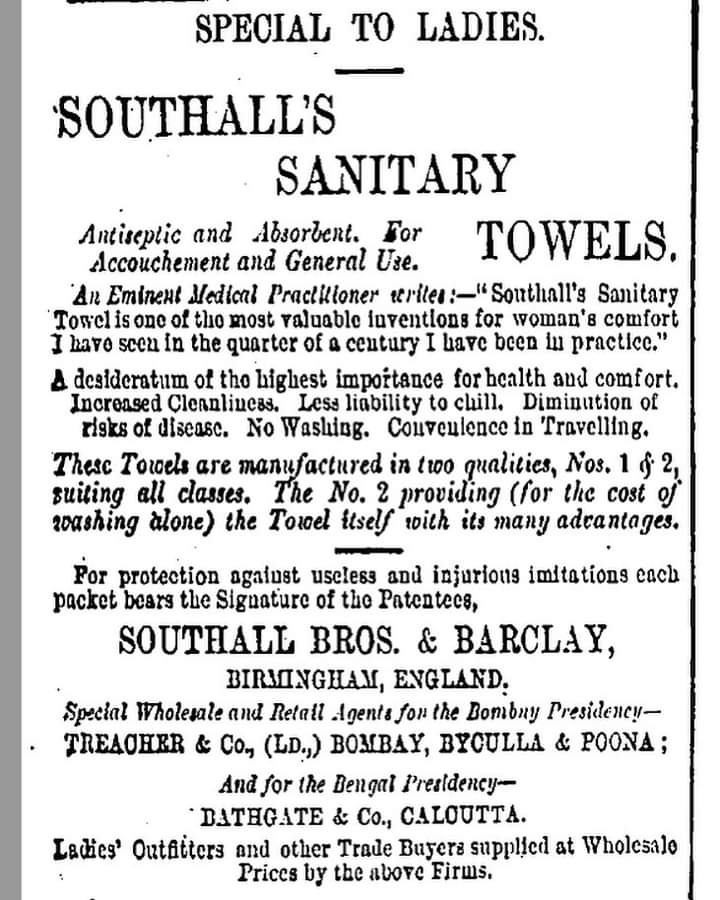The image depicts an old newspaper clipping, mostly in shades of white, black, and gray, that takes up the entirety of the photo. The text is centered and formatted vertically, highlighting an advertisement for Southall Sanitary Towels, described as antiseptic and absorbent, designed for accouchement and general use. The advertisement features a testimonial from an eminent medical practitioner, stating that these towels are one of the most valuable inventions for women's comfort he has seen in his 25 years of practice. The testimonial emphasizes their importance for health and comfort, including benefits such as increased cleanliness, reduced liability to chill, decreased risk of disease, and the convenience of not requiring washing. The towels are available in two qualities to suit all classes, with the second grade intended as a cost-effective option. Each packet is protected against imitation by bearing the signature of the patentees, Southall Brothers and Barclay from Birmingham, England. The clipping also lists special wholesale and retail agents for different regions, including Treacher and Company in Bombay, Byculla, and Puna, and Bathgate and Company in Calcutta.